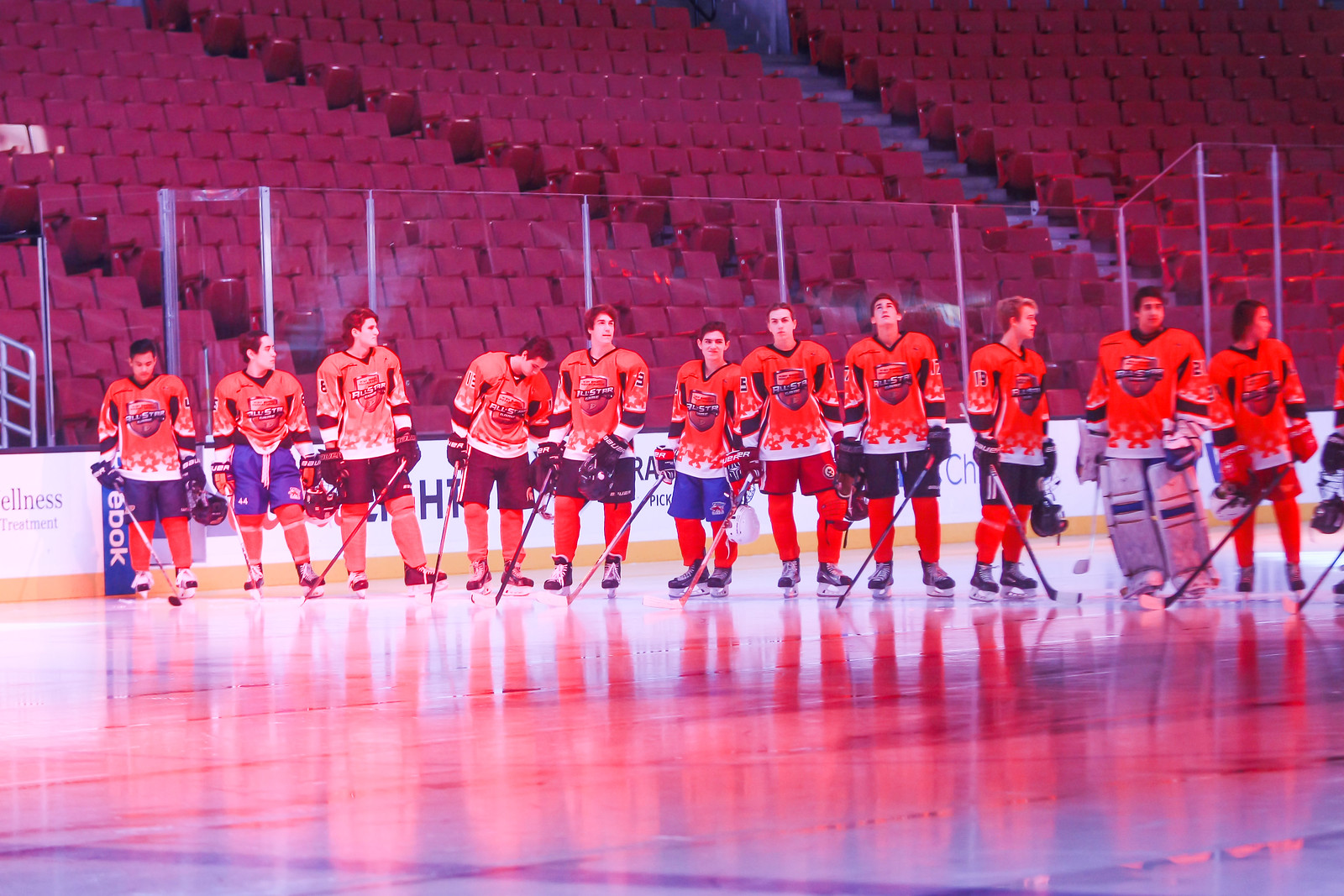The indoor photograph captures an ice hockey team posing on a pristine, reflective ice rink. The team consists of eleven players lined up, most facing toward the camera, dressed uniformly in red jerseys with blue pants, and some differing in shorts color. Their reflections cast red and blue hues on the ice surface. Notably, the second player from the right, identifiable as the goalie, wears distinctive leg guards. The team stands before a plexiglass barrier, which serves to protect the audience during gameplay. Beyond the barrier, the empty stadium seats stand out in vivid red, with white staircases and railings interspersed among many rows, accentuating the detailed, layered backdrop. The scene is lit with a soft, red hue, adding a harmonious tone to the overall image.